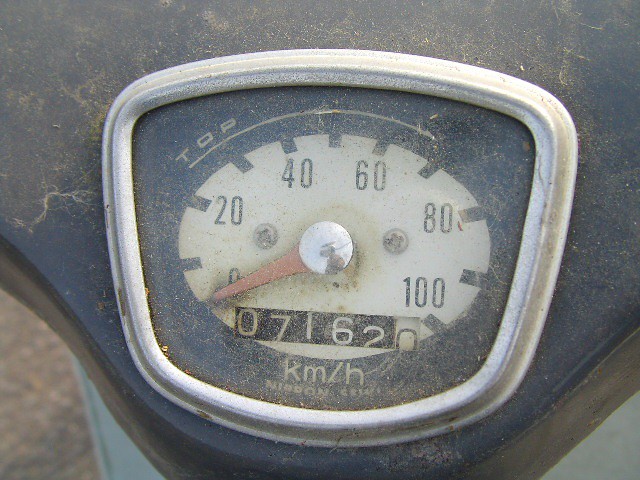Close-up of an old-style speedometer from a vintage bike, framed with a metallic rim and mounted on dirty black handlebars. The image zooms in tightly on the almost rectangular device with rounded edges. The dial, a mix of white and black, marks speeds from 0 to 100 kilometers per hour, with large numerals at 20-kilometer intervals. At its center, a shiny chrome circle reflects light, anchoring the red needle that points out the current speed. The mileage reads 071620 kilometers, hinting at the bike's extensive use. Dirt covers much of the speedometer, blurring the glass but leaving the numbers visible, while a bit of the rough road surface peeks through at the bottom, emphasizing the outdoors setting.